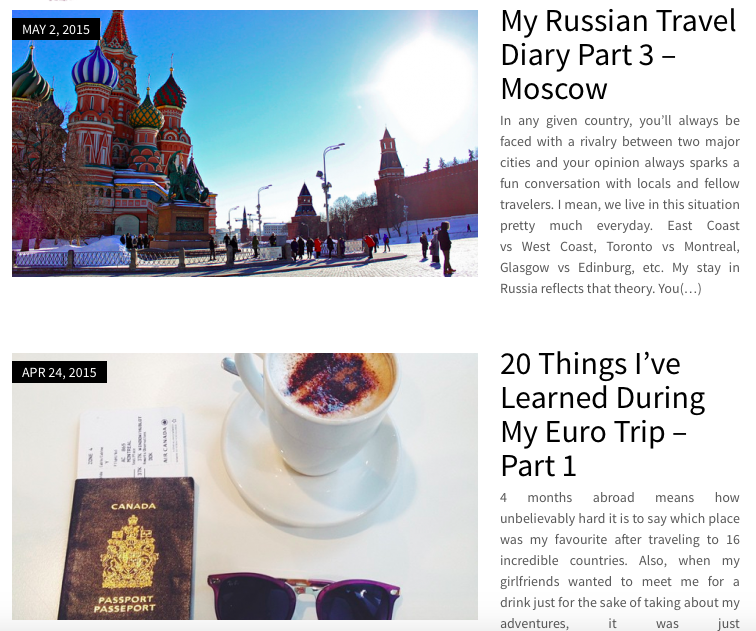This image is a screenshot of a travel diary, possibly part of a travel blog. The diary entries are visually documented, with the first one dated May 2, 2015, titled "My Russian Travel Diary, Part 3: Moscow." This entry includes a photograph depicting Moscow, highlighting some downtown area with several buildings in the background. The second diary entry is dated April 24, 2015, and is labeled "20 Things I've Learned During My Euro Trip, Part 1." Accompanying this entry is a photograph featuring a cup of coffee, a pair of sunglasses, and a Canadian passport, which holds what appears to be a boarding pass inside.